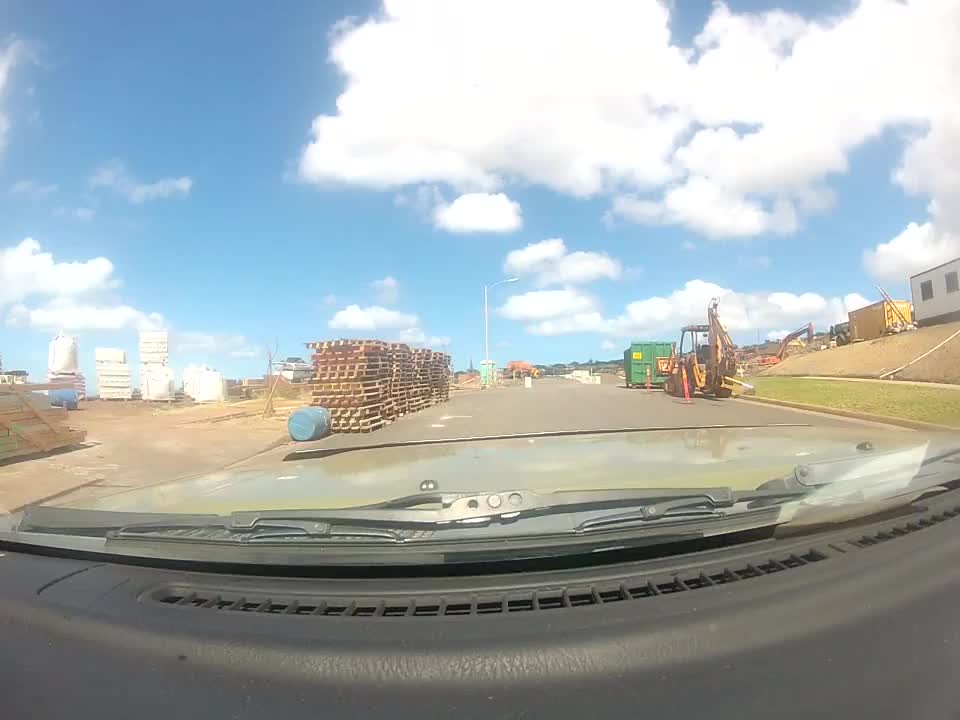A high-resolution dash cam captures a sleek car speeding down an unfinished residential development, reminiscent of scenes from "Fast and Furious: Tokyo Drift." The housing structures, still under construction, create a dynamic backdrop as the vehicle blurs through the debris and scaffolding, evoking the high-octane action sequences iconic to the film. The setting's raw, half-built aesthetic contrasts sharply with the vehicle's modern design, amplifying the sense of adrenaline and urgency in the moment.